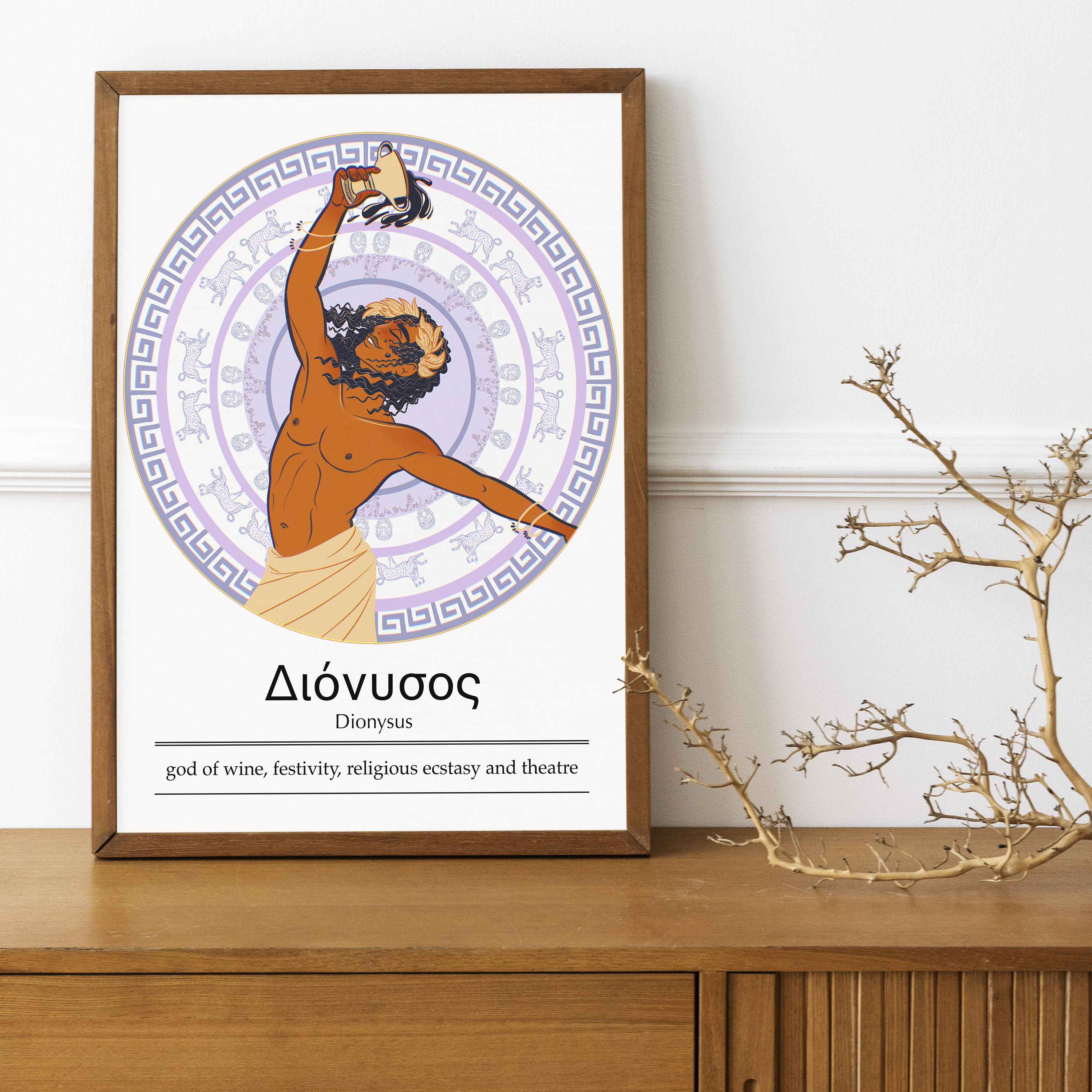The image depicts a detailed scene centered around a Greek-themed depiction of Dionysus, the god of wine, festivity, religious ecstasy, and theater. The main focus is a framed illustration resting on a light brown credenza or buffet. The wooden frame encases a white background featuring a muscular man with tan skin, black wavy hair adorned with flowery bits, and a white toga wrapped around his lower half. He is holding a beige chalice at the top of his head, from which black liquid pours out. Behind him, there's a Greek concentric circle design and purple accents, contributing to the mythical ambiance. On the wooden surface to the right, there's a leafless tree branch. The background wall is plain white, highlighting the overall Greek god motif. The inscription beneath the image reads: "Dionysus, god of wine, festivity, religious ecstasy, and theater."